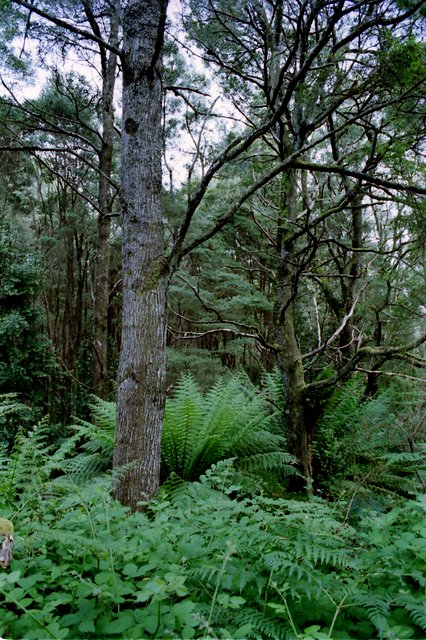The photograph captures a dense, possibly damp forest with a tall, grayish tree positioned center-left, notable for its thickness and several protruding limbs, all barren of leaves. On the center-right, there's a thinner tree with multiple limbs, also leafless. The background is filled with taller trees adorned with green leaves, adding depth to the scene. In the foreground, vibrant green fern plants and berry bushes cover the ground, contributing to the lush undergrowth amidst which a pine tree with green moss and some dead branches stands. The atmosphere appears humid and overcast, with a mostly gray sky peeking through the dense foliage, indicative of a cloudy day. The photo, likely taken with a camera phone and vertically oriented, showcases the forest's layered composition, from the rich foreground flora to the towering, leafy trees in the distance.